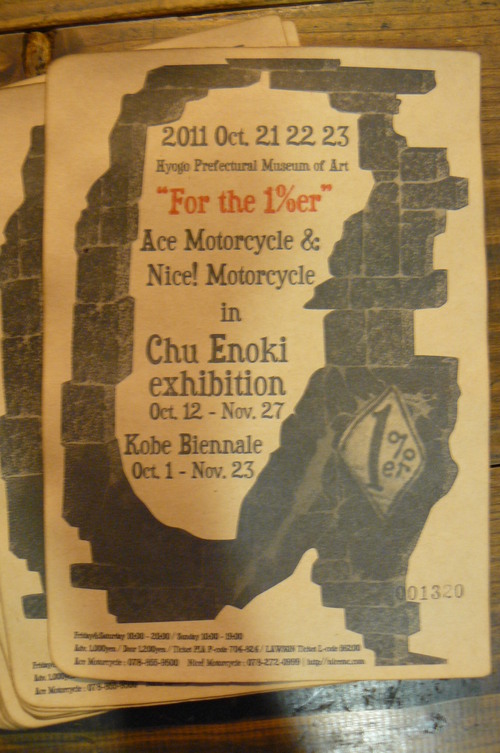The image depicts a weathered, vertically rectangular advertisement flyer for a 2011 motorcycle-themed art exhibition. The flyer, printed on dirty white paper, is affixed to a wooden wall, overlapping other identical posters on the left side. The central feature is a semi-circular brick motif encircling the event details in the middle. The prominent text reads, "2011, October 21st-23rd, Hayug Prefectural Museum of Art for the 1%er," likely referring to a motorcycle gang. It announces the Ace Motorcycle and Nice Motorcycle in Chu Enki Exhibition from October 12th to November 27th, and the Kobe Biennale from October 1st to November 23rd. The bottom of the poster contains fine print that's too small to read clearly and a unique identification number: 001320. The color scheme includes black, off-white, brown, beige, and red. Additionally, a small sticker or patch with "1%er" is affixed to the brick outline on the right. The photograph captures the scene indoors, showing the flyers upright on a wooden surface. Despite being labeled "2011," the flyer appears considerably older.